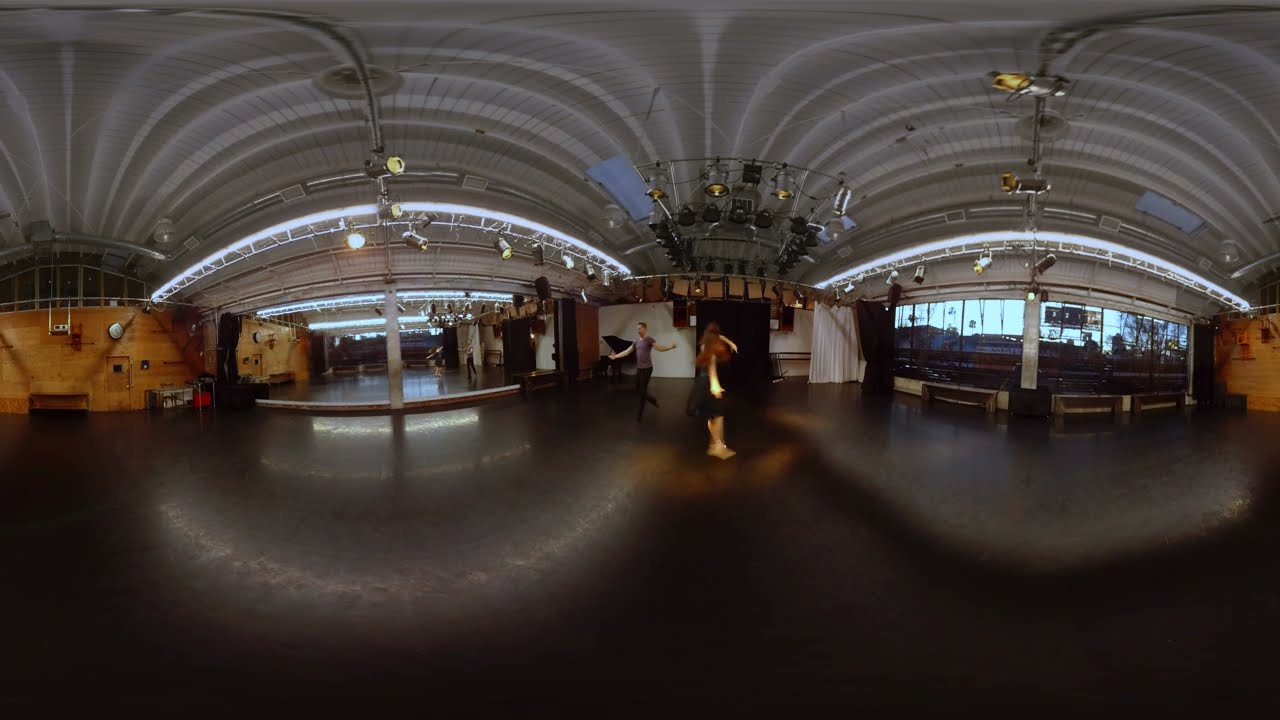The image depicts a spacious, indoor, warehouse-like dance studio with a smooth, shiny, dark brown-blackish reflective floor and a lighter gray ceiling filled with various can lights pointing in different directions. The setting appears to be a large, mostly empty room with minimal furniture, save for some benches, allowing ample space for movement. This 360-degree panoramic photograph, which slightly distorts some lines, features a couple dancing at the center: a male dancer in a purple shirt and black pants, standing with his arms by his side, and a woman dressed in a flowing attire dancing away from him. The studio's layout includes a substantial mirror on one wall and large windows on another, which provide a view of the outdoors, suggesting the time might be nearing evening, as it appears somewhat dim with both indoor and outdoor lights on. There are also wooden walls and a doorway leading outside seen in the far end of the image. Additionally, some scaffolding or a catwalk-like structure with lights is mounted on or near the ceiling. The overall ambiance feels bright yet tranquil, underscored by the rarity of other people in what is a broad and open area.